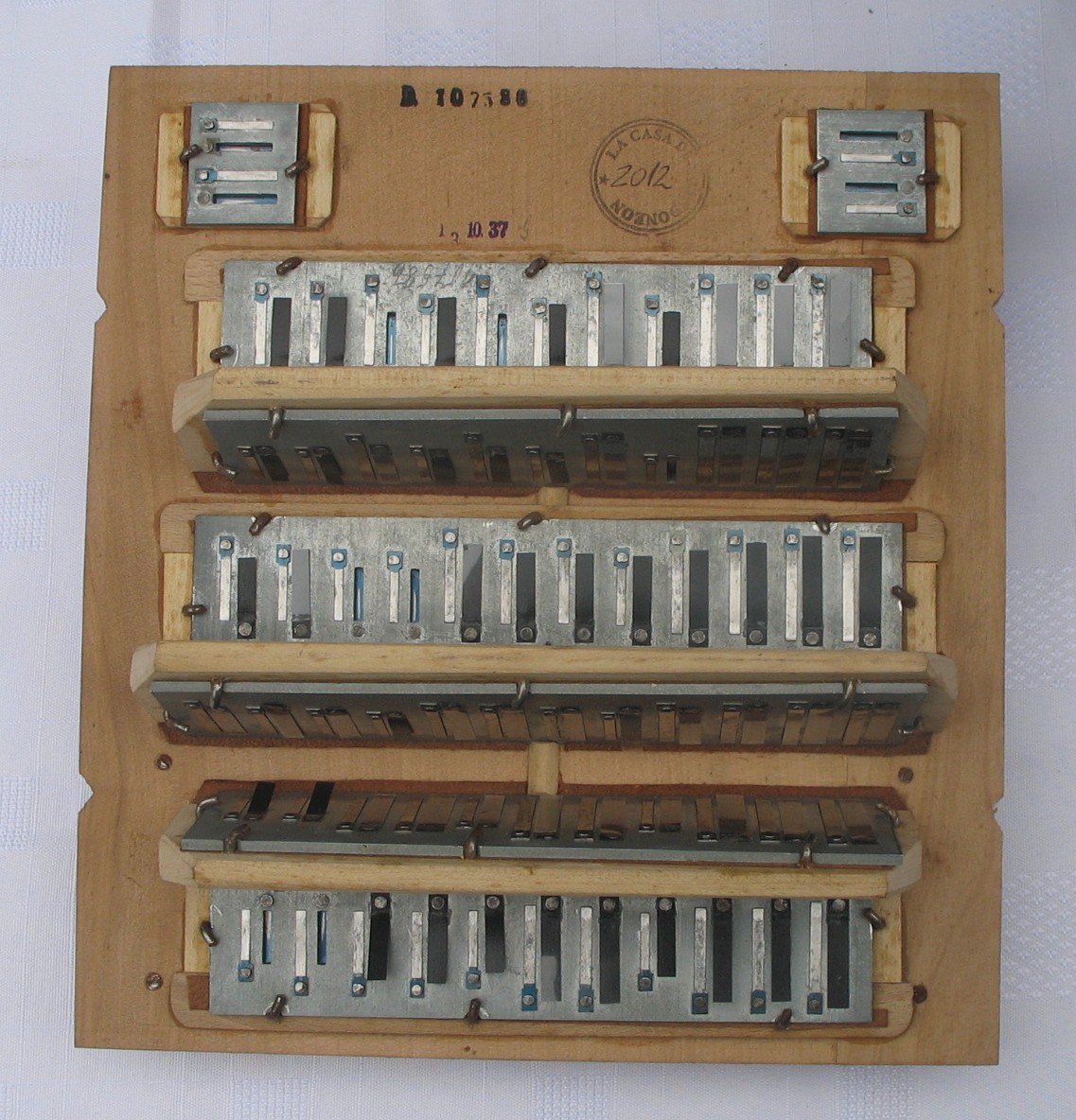The photograph depicts a vertical rectangular wooden panel, made of thin plywood, set against a white background with various metallic attachments. At the top of the panel, the number "107586" is stamped in black ink. Below this stamp, on the right side, there is a circular postmark-like stamp that reads "La Casa De" at the top and includes the handwritten year "2012" in the center, though the rest of the text within the circle is illegible.

The main feature of the panel consists of three horizontal metal panels or slats with vertical black rectangular slots. These metal panels are arranged in three rows, attached to the wooden surface. Additionally, there are two small square metal areas positioned at the upper left and upper right corners of the panel. Each of these components appears securely fastened with small metal attachments. The metal slats feature small vertical strips, some white with blue squares at the top, and some black, possibly with circular silver elements at their ends. The precise function of these metal and wood structures is unclear, but they resemble shelving or support elements, creating an intricate and organized layout on the wooden board.